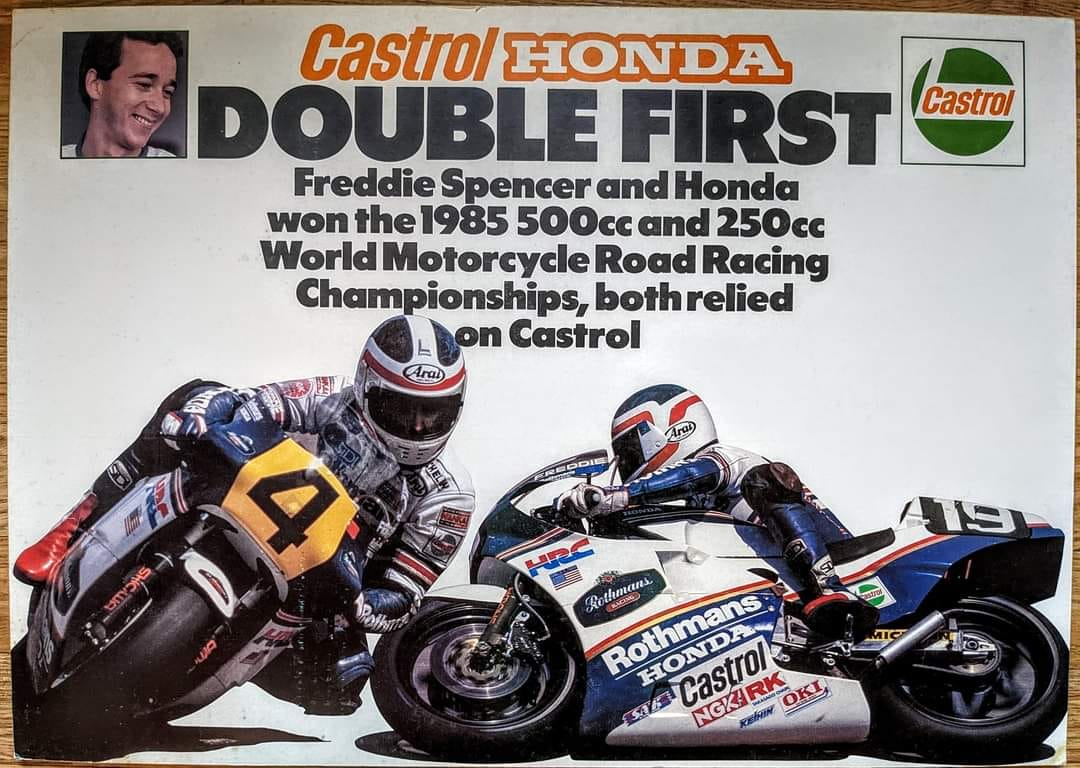This is an advertisement poster for Castrol Oil, featuring the "Castrol Honda Double First" racing event. The background is white, and prominently displayed at the top is the text in orange: "Castrol," next to "Honda" in white print outlined in orange. Below is the bold, black, all-capitalized text: "DOUBLE FIRST."

The poster celebrates the achievements of Freddy Spencer and Honda, who won the 1985 500cc and 250cc World Motorcycle Road Racing Championships, both relying on Castrol. There are two dynamic images of motorcycles: one (number 4) is tilting around a curve, headed toward the camera, showcasing its aerodynamic fairing and sponsor decals, and the other (number 19) is displayed from a side view.

On the top left corner of the poster is a square photograph of a man with short dark hair, dark eyes, and a contemplative gaze. On the top right corner is the Castrol logo, within a white box outlined possibly in green or black.